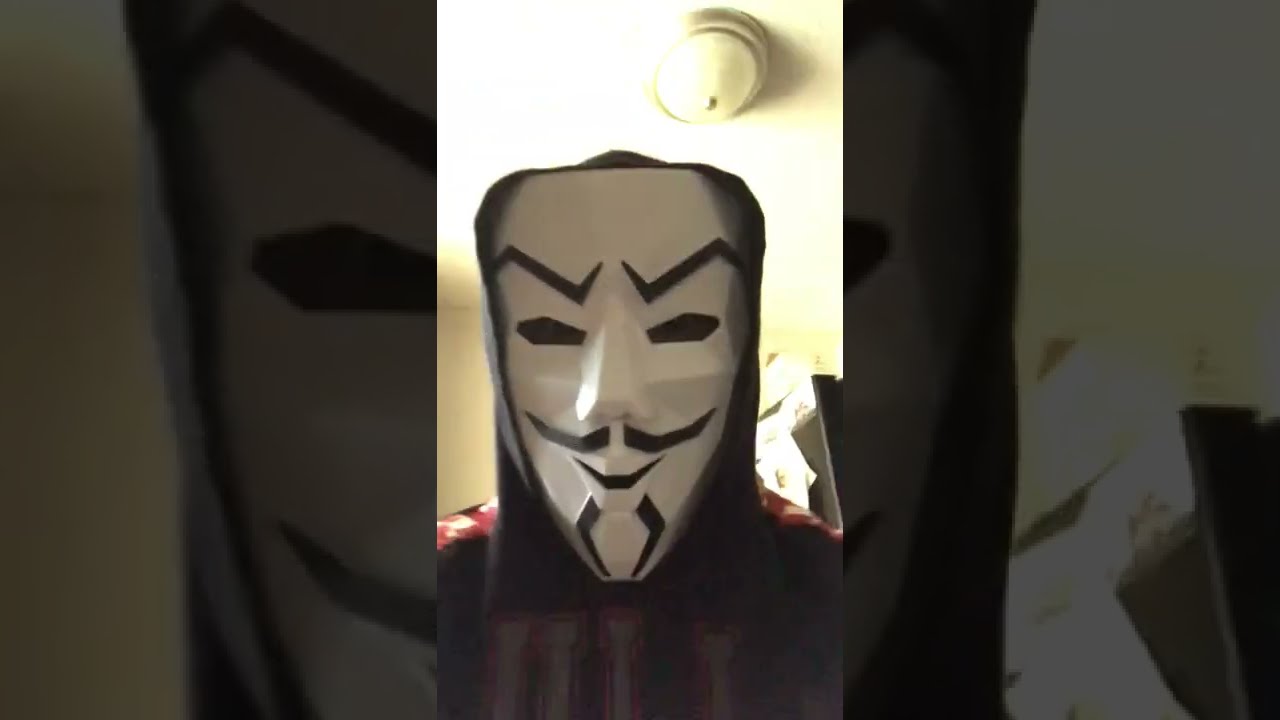This image features a split composition divided into three parts, with the central section being the main focus. In the center, a person is wearing a striking white and black mask, which appears to be plastic with a sinister design. The mask showcases black, oval-shaped eyes, and angular, jagged eyebrows forming a Z-like shape. It features a detailed mustache extending thinly to the sides, a slightly open, black smile, and two lines forming a goatee beneath the lips. The person is also dressed in a black hoodie adorned with white lettering bordered in red and a design of red and white stripes on the shoulders. They are situated indoors, under a white ceiling with a circular light fixture visible above them, which could be a smoke alarm or a bulbous light. The left and right sections of the image display darker, close-up views of the same masked face, framing the central portrayal and emphasizing its details.